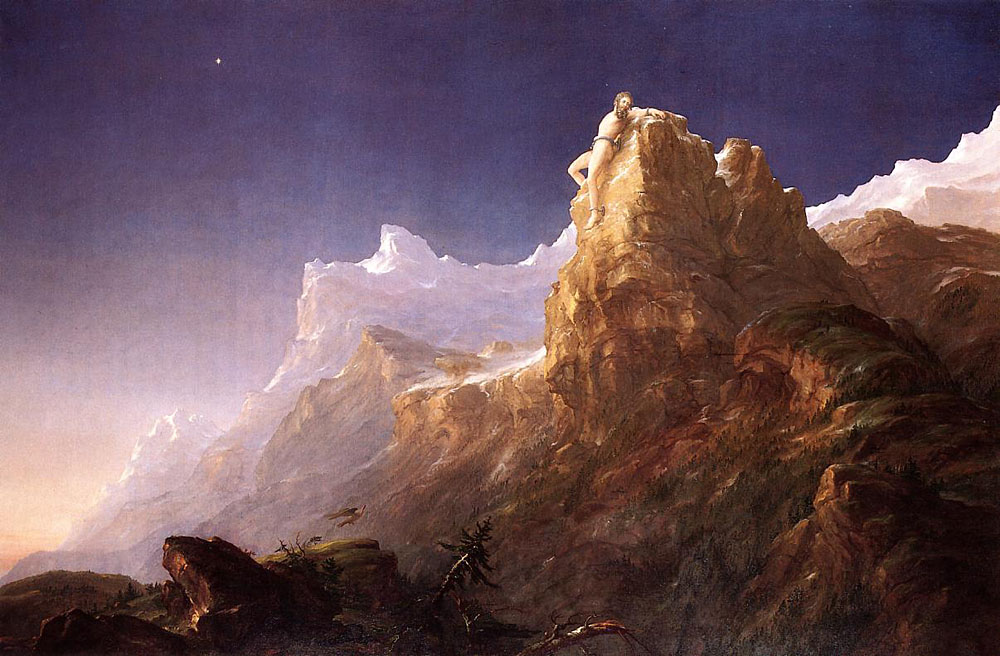The painting depicts a dramatic and surreal scene of a nearly naked man clinging desperately to a sheer, craggy cliff face that rises steeply above a canyon. His back is pressed awkwardly against the rugged brown and orange rock, and his head is tilted back as he looks upwards in a seemingly impossible position, suggesting a struggle for survival. The cliff itself features sparse, dark rocky terrain in the foreground, with a few spindly tree trunks jutting out. Above, the scene transitions into a vividly colored sky—blue at the zenith, blending into hues of orange indicative of either sunrise or sunset. This majestic backdrop includes hints of jagged, icy white snow-capped peaks or possibly clouds. The figure's ordeal is set against this backdrop of distant mountainous ranges, giving the entire image an ethereal and poignant touch with a single star visible in the sky. His arms appear outstretched as if impaled or bound to the rock, evoking a crucifixion-like pose that further emphasizes the intense, almost sacred struggle depicted in this enigmatic and haunting artwork.